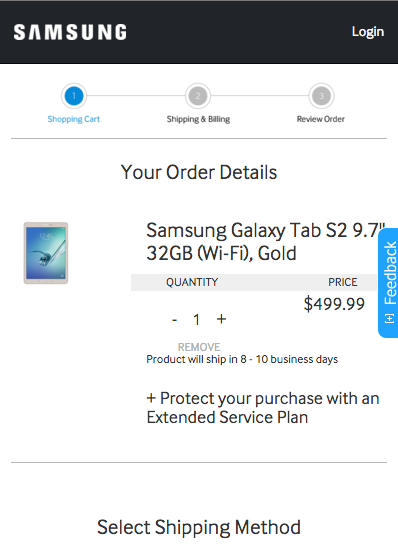This screenshot captures a detailed view of a Samsung shopping website. At the top, a solid black banner features bold, white block text. In the upper left corner, "Samsung" is prominently displayed in their iconic font, while the upper right corner has the word "Login" in white text. Below the banner, the page layout indicates it is a shopping site, with a blue-highlighted circle on the left labeled "1. Shopping Cart," connected by a gray line to the next steps: "2. Shipping and Billing," and "3. Review Order."

Underneath these steps, a thin gray line stretches horizontally across the page, followed by a large black text header that reads, "Your Order Details." Below this header, specifics of the purchase are listed: a Samsung Galaxy Tab with a 29.7-inch display, 32 gigabytes of storage, Wi-Fi capabilities, in gold color. The quantity is noted as one, and the price is set at $499.99. To the left of this information, there is a color image of the product, showcasing the tablet. Below the product description, there is an option to enhance the purchase with an extended service plan, indicated by a plus sign.